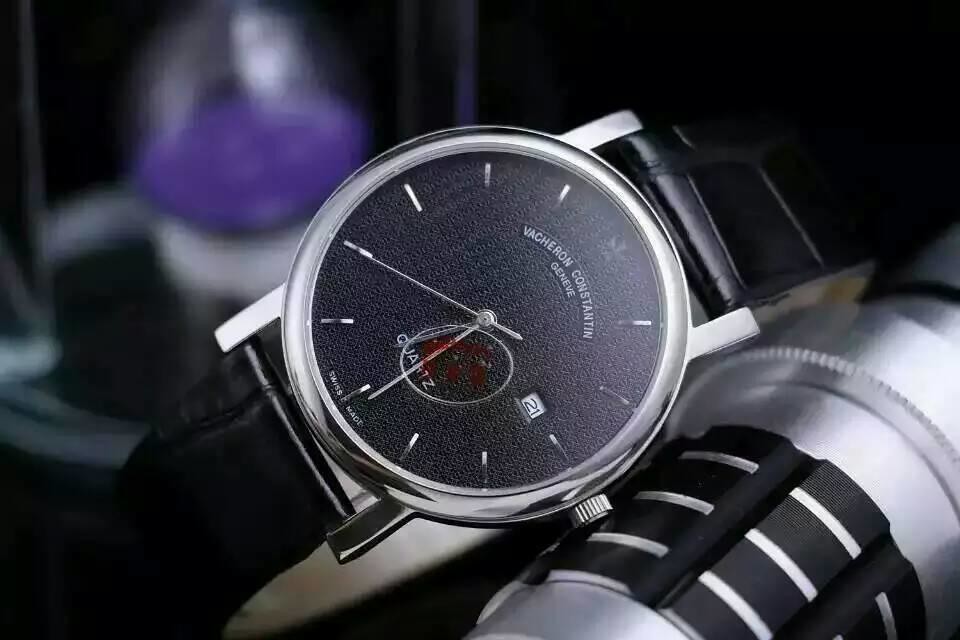The image depicts a black wristwatch with a sleek black strap and a black face, surrounded by a silver bezel. The watch features minimalist hour markers, consisting of silver lines instead of traditional Roman numerals. The watch hands are silver, and an engraving on the watch reads "Veterans Consenting Courts." The current time displayed is 5:40. Beside the watch is a stainless steel tumbler, possibly a thermos, adorned with black accents. The items appear to be placed inside a car, suggested by a visible drink holder in the background on the left side, which is black and holds a small plastic cup with an unidentified object on top.